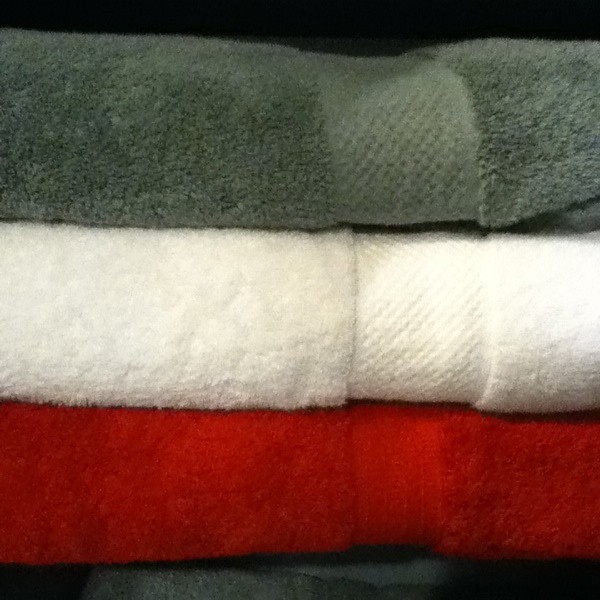The photo showcases four plush, neatly stacked towels against a black background, which is visible only as a narrow strip at the top. The towels are folded or rolled up, appearing soft and fluffy, each featuring a distinctive compressed stripe texture toward the right side. The top and bottom towels are of a greenish-bluish-gray color, while the middle ones consist of a bright white towel followed by a deep red towel. Only partial sections of the towels are visible due to the close-up framing, giving a detailed view of their plush texture and tidy arrangement.